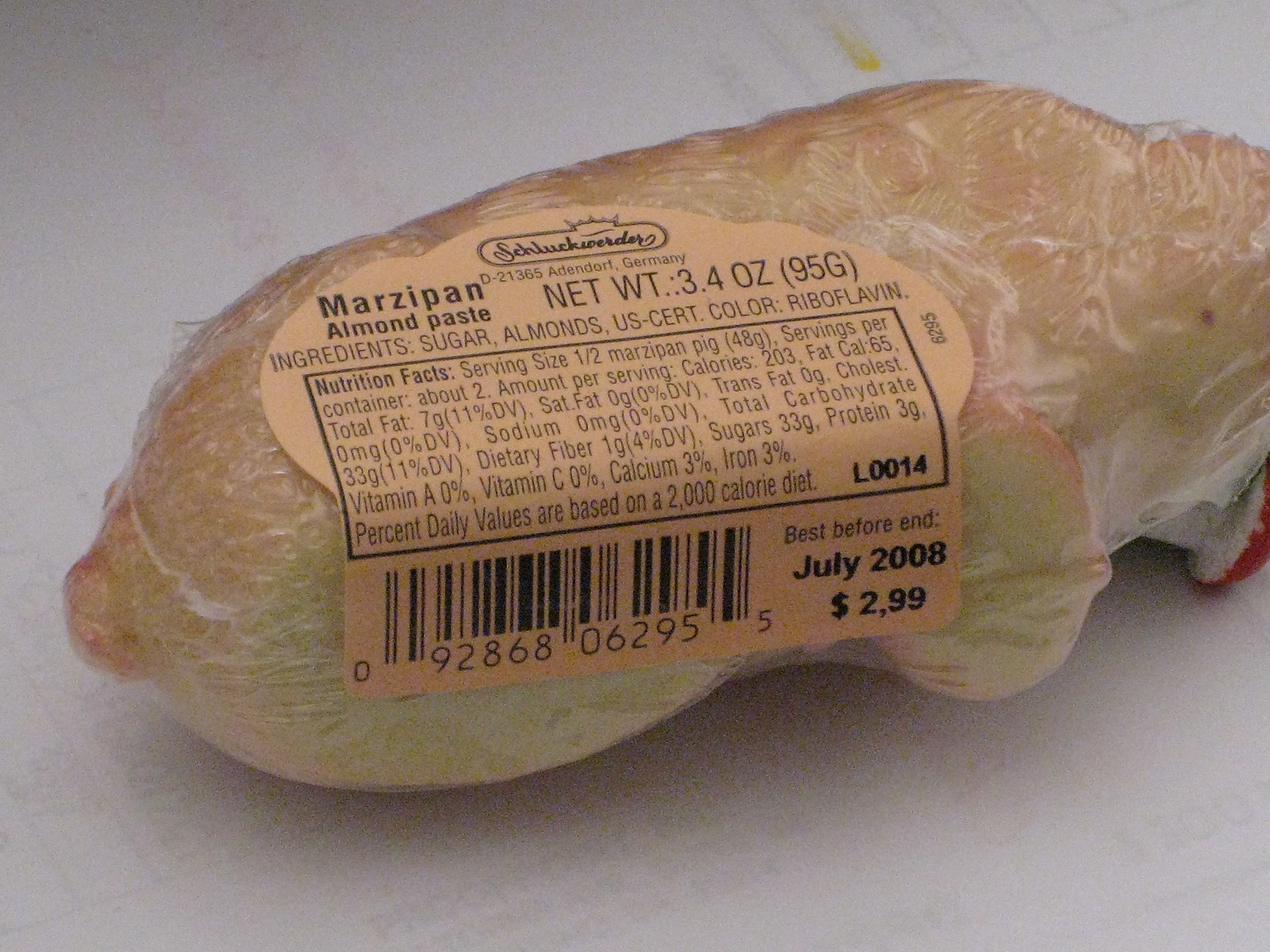This image features a close-up view of a package of marzipan almond paste. The marzipan is tightly wrapped in clear plastic, showcasing its dense, beige texture. A peach-colored label affixed to the packaging provides a comprehensive list of ingredients, nutritional facts, and other pertinent information. The product is priced at $2.99 and has a "Best Before" date of July 2008. The label, slightly faded but still legible, indicates that the marzipan paste weighs 3.4 ounces. Additionally, a barcode (UPC) is displayed at the bottom of the label. The paste is noted to be manufactured in Germany, though the company logo present is challenging to decipher.